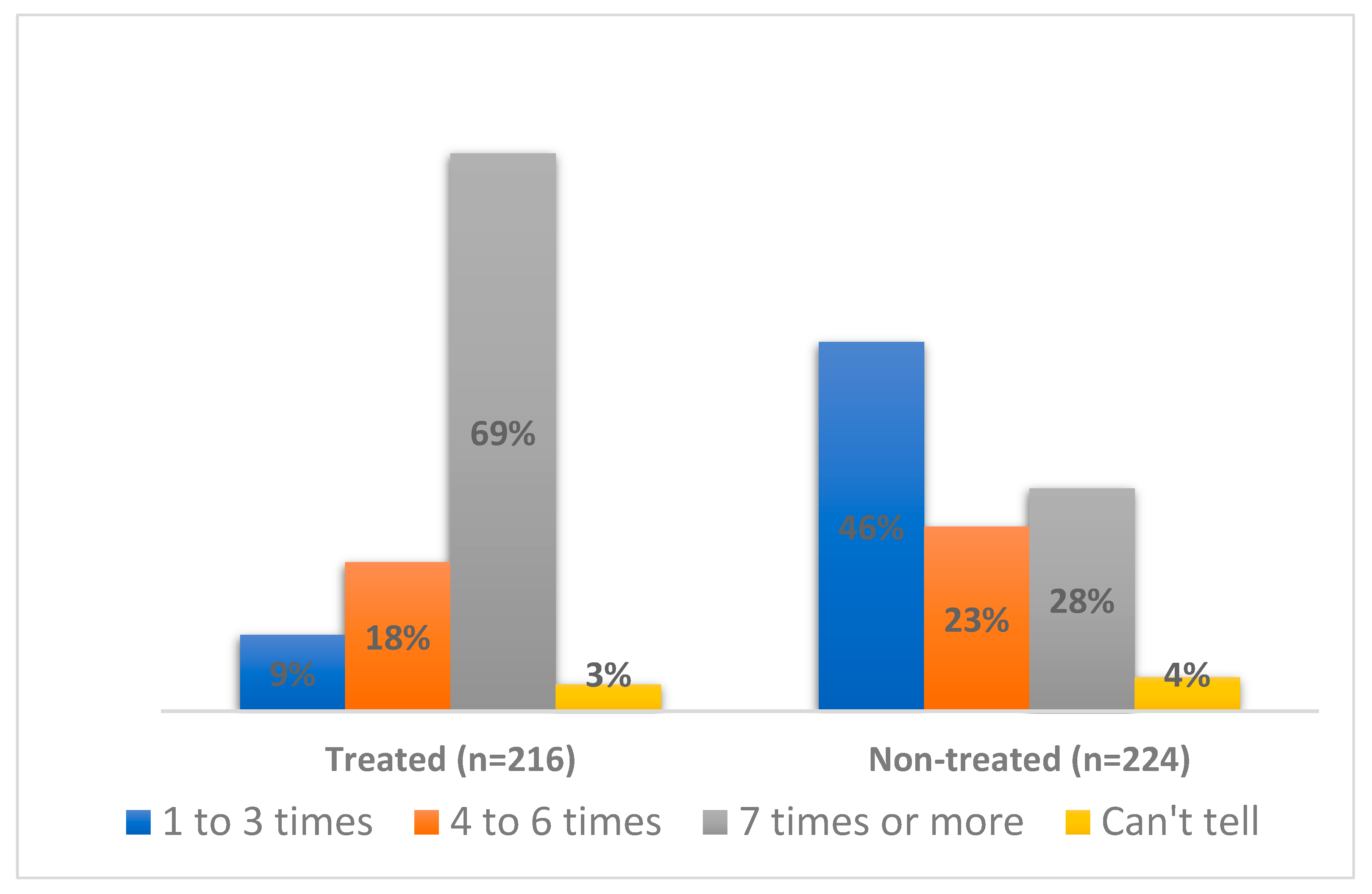The image depicts a detailed bar graph with a white background and a thin gray line outlining the graph area. The graph compares two conditions: "treated" (left side, N=216) and "non-treated" (right side, N=224). Each side contains four bars, distinguished by different colors according to a legend at the bottom: blue (1 to 3 times), orange (4 to 6 times), gray (7 times or more), and yellow (can't tell).

In the treated condition, the bars represent:
- Blue: 9% (1 to 3 times)
- Orange: 18% (4 to 6 times)
- Gray: 69% (7 times or more) 
- Yellow: 3% (can't tell)

The non-treated condition shows:
- Blue: 46% (1 to 3 times)
- Orange: 23% (4 to 6 times)
- Gray: 28% (7 times or more)
- Yellow: 4% (can't tell)

Each color corresponds to the frequency of an unspecified treatment, with the gray bar being the tallest in the treated group and the blue bar being the tallest in the non-treated group.